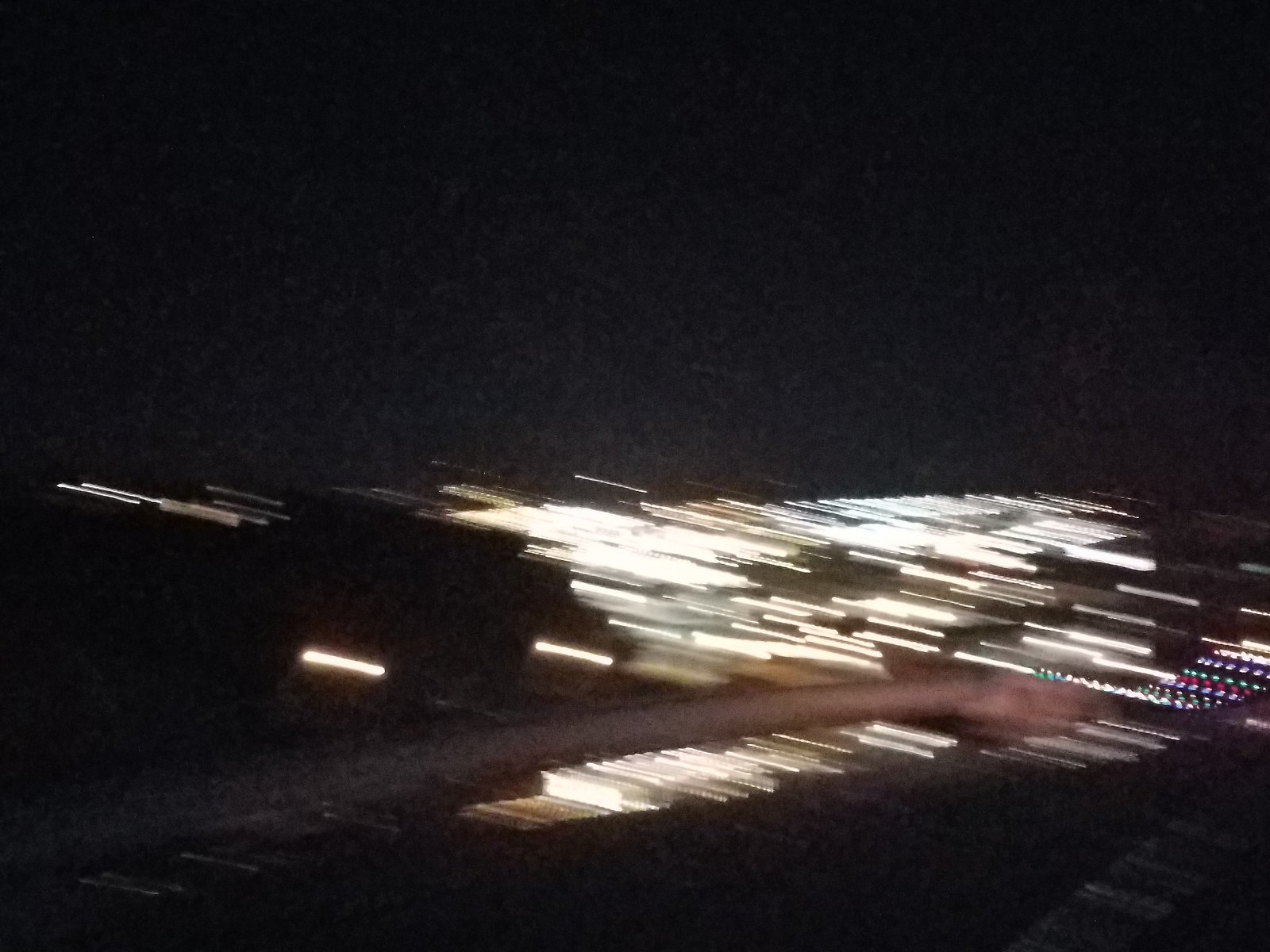This photograph appears to be an aerial shot, possibly taken from an airplane during take-off or while in flight. The image is extremely blurry, dominated by darkness with a predominantly black background. The most discernible feature is a network of bright white lights, some of which are dotted with greens, reds, and blues, mostly situated towards the bottom right and a bit in the center of the image. The arrangement and motion of these lights suggest movement, almost as if they are vehicles on a highway or city streets, or the lights of a flying vehicle like an airplane. Additionally, near the bottom right, there's a vague shape that could either be a roadway, an abstract reflection, or even part of the airplane itself, though this detail remains indistinct. Overall, the photograph captures an impression of luminous trails against a dark backdrop, evoking a sense of motion and the night-time urban or aerial landscape.